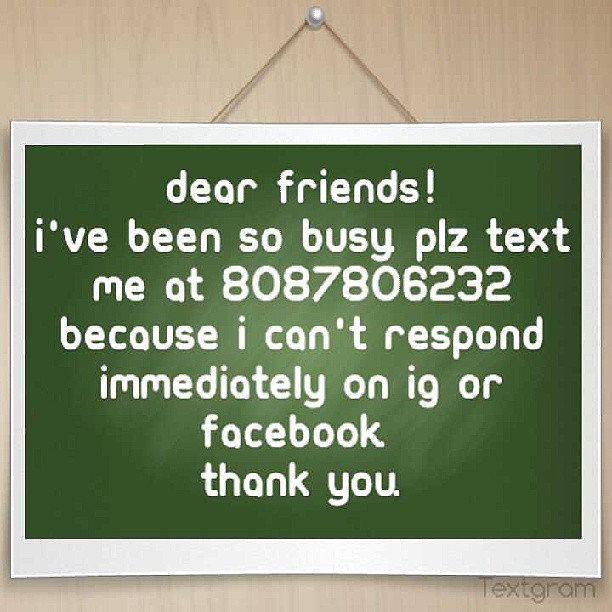This is a detailed digital image resembling a notice board. The image has a light tan background designed to look like a wall, with a silver tack at the top center, resembling a pearl-capped thumbnail. From this tack, brown strings angle downward in a triangular fashion to hold up a digitally crafted sign. The sign itself is horizontally rectangular, with a dark green center and a white border surrounding it. Written in white text on the green background are the words: "Dear Friends! I've been so busy. Please text me at 808-780-6232 because I can't respond immediately on IG or Facebook. Thank you." At the bottom right corner of the sign is a watermark that reads "Textgram." The entire image, though digitally rendered, effectively simulates a physical notice pinned on a wall.